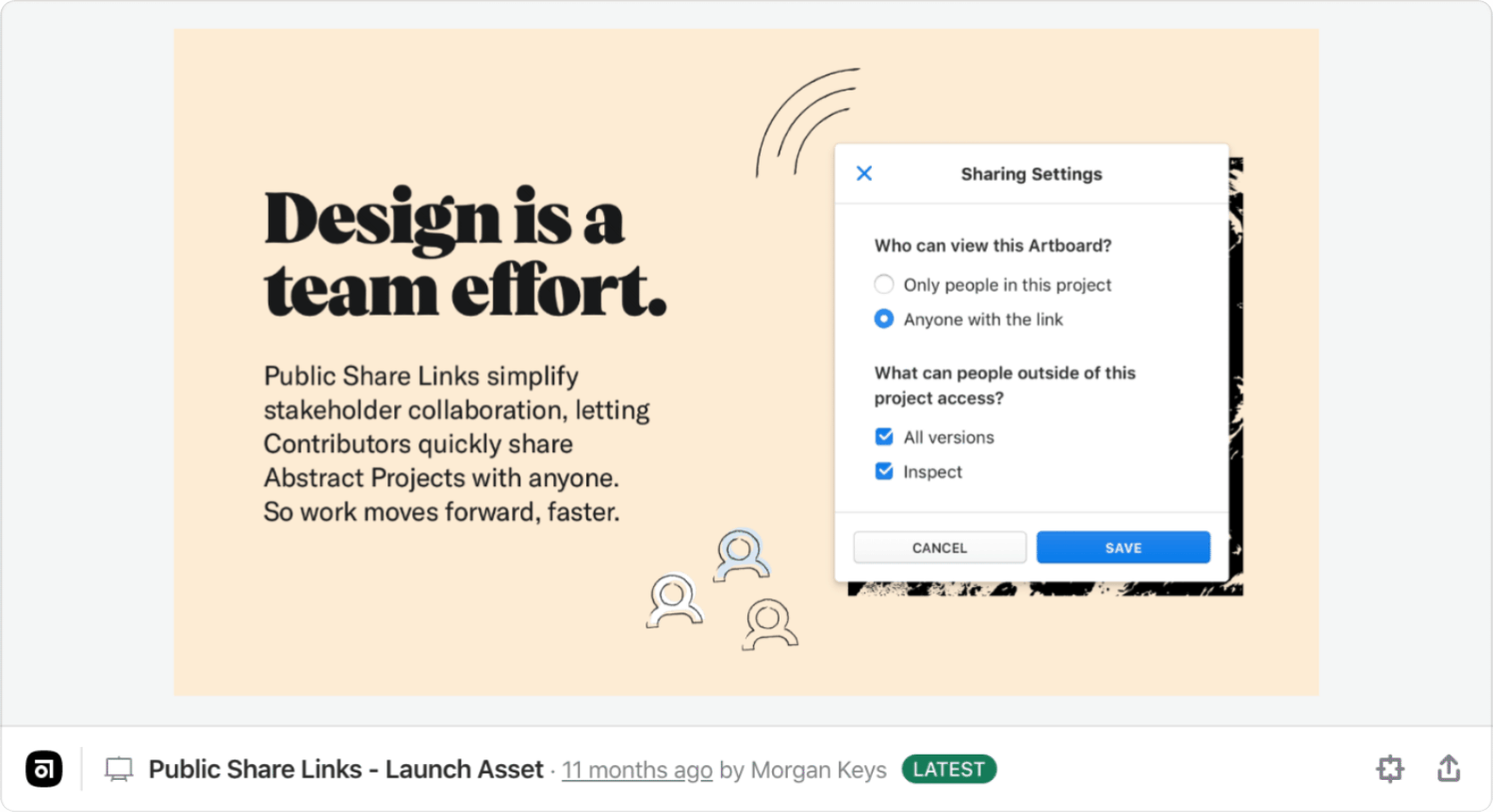This image features a digital screenshot displayed against a white background. Central to the screenshot is a light gray rectangular box bordered by a tan rectangular box on the left, housing dark brown text. The text reads, "Design is a team effort," in lowercase, smaller font. Below this, a more substantial block of text states: "Public share links simplify stakeholder collaboration, allowing contributors to quickly share abstract projects with anyone. This accelerates project progress."

To the right of this text, a smaller white box includes the label "Shared Settings." Underneath, a highlighted blue option inquires, "Who can view this artboard?" with options marked for “Only people in this project” or “Anyone with the link,” the latter being circled in blue.

Below this are permissions settings, asking, "What can people outside of this project access?" with checked boxes for “All versions” and “Inspect.” Directly beneath these options are two buttons; a white one labeled "Cancel" and a blue one labeled "Save."

On the lower left side of the screenshot, there’s an icon resembling a computer monitor. Just below the icon, text reads: "Public share links launch asset 11 months ago by Morgan Keyes."